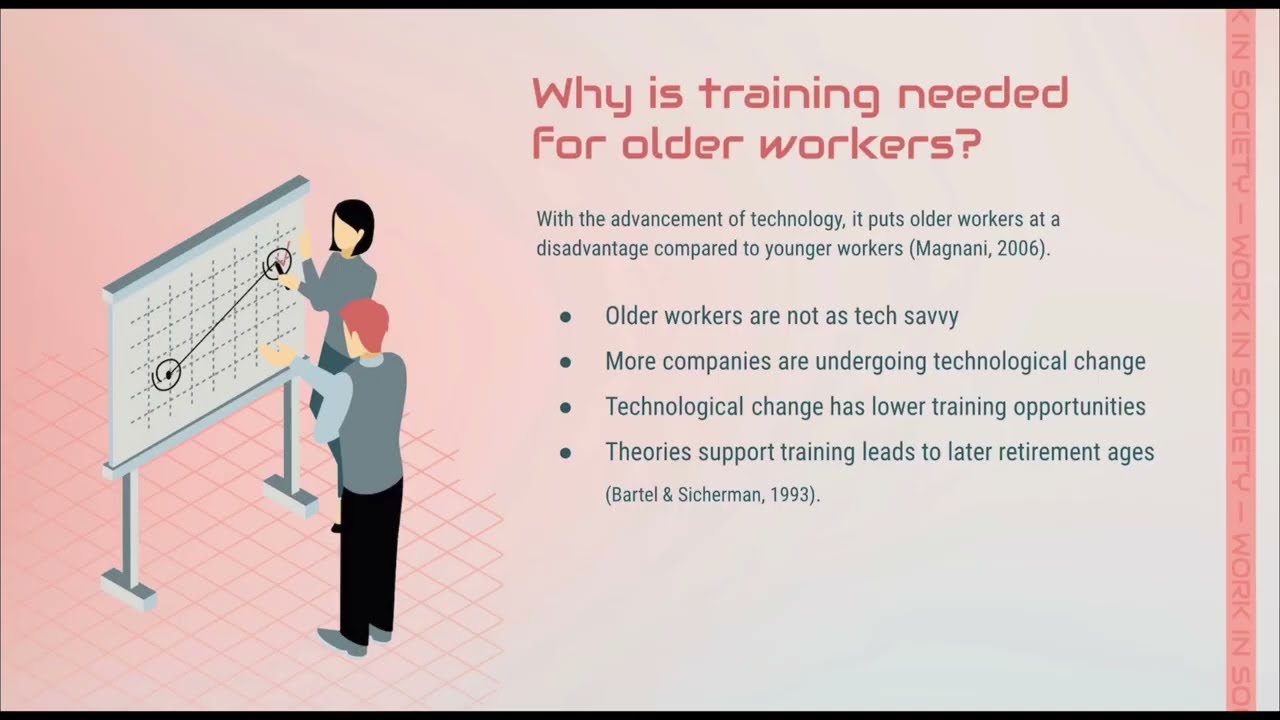The image is an illustrative slide from a presentation with a pale peach to gray gradient background, featuring black headers and footers. The central visual elements include two clip art characters without facial features—a woman with dark hair who appears to be explaining a chart, and a man with red hair who is gesturing towards the chart. The chart, mounted on a whiteboard with grid lines and standing on steel legs, depicts a simple diagram with two interconnected circles.

To the right of the characters, the slide title in red text reads, "Why is training needed for older workers?" Directly below, in blue text, a subheading states, "With the advancement of technology, it puts older workers at a disadvantage compared to younger workers (Magnani, 2006)." This is followed by four bullet points: "Older workers are not as tech savvy," "More companies are undergoing technological change," "Technological change has lower training opportunities," and "Theories support training leads to later retirement ages (Bartel and Sickerman, 1993)."

A vertical peach stripe on the far right of the slide displays the repeated text "Work in society." The style of the image is both informative and illustrative, designed to visually communicate the necessity for training programs targeted at older workers amidst technological advancements.